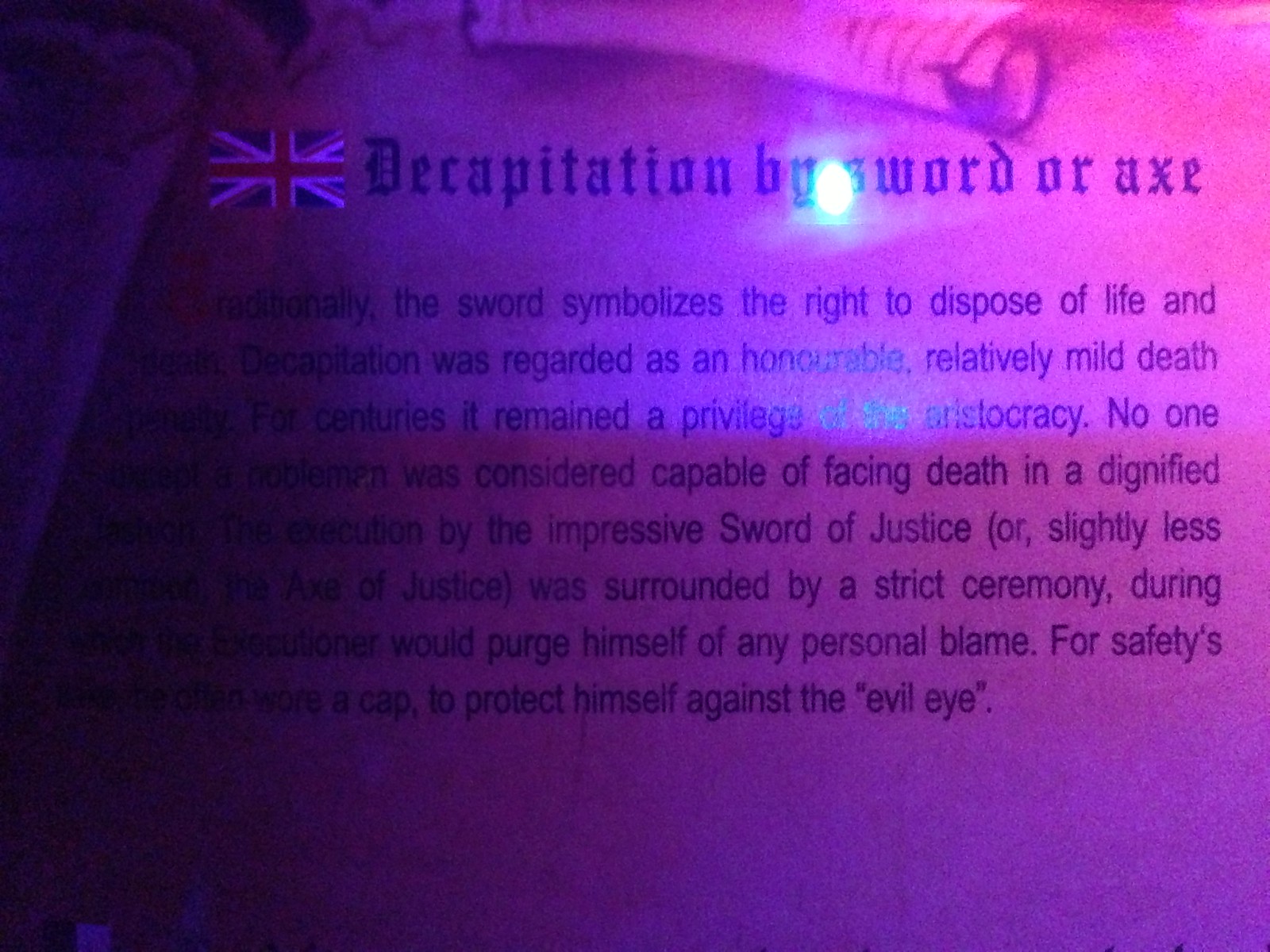This image appears to be a poorly taken photograph of an explanatory plaque or a book page, tinged with a purplish hue and featuring a reflective glass cover, making it difficult to read. It shows a section shadowed and out of focus, with the right-hand portion more legible but lacking full context due to the obscured left-hand side. The title, "Decapitation by Sword or Axe," written in an Old English font, is accompanied by an image of the Union Jack in the top left corner, indicating its British context. The available text describes how decapitation was historically viewed as an honorable and relatively mild form of death, traditionally reserved for the aristocracy, and was surrounded by strict ceremonial practices. Notable phrases explain how the "sword of justice" was employed, and how executioners would wear a cap to protect themselves against the "evil eye," attempting to purge any personal blame. The overarching theme relates to the medieval British practices of execution, emphasizing the ceremonial and societal perceptions of decapitation.